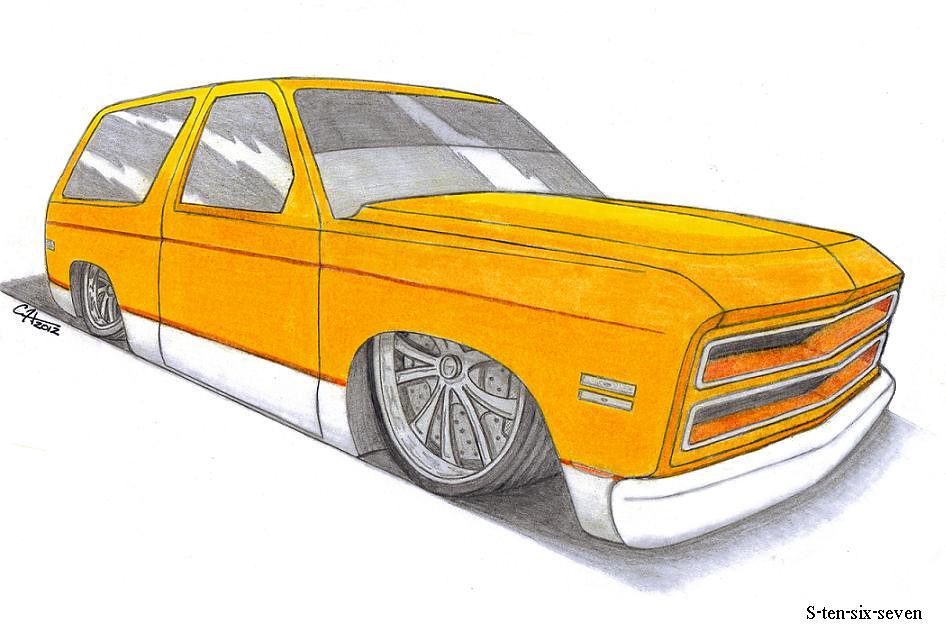The image features a detailed color drawing of a car with a yellow, slightly orange body and white accents on the bumpers and side skirts. The gray windows show light reflections through lighter sections. At the front, the car has two long horizontal grilles instead of headlights. The wheels, detailed with large rims, are recessed into the chassis, giving the impression that the bottom of the vehicle is touching the ground. The car is labeled with the text "S1067" at the bottom. The background of the image is white, with a subtle drop shadow beneath the car. The drawing takes up the bottom right corner and positions the car facing from the upper left to the middle right of the image.